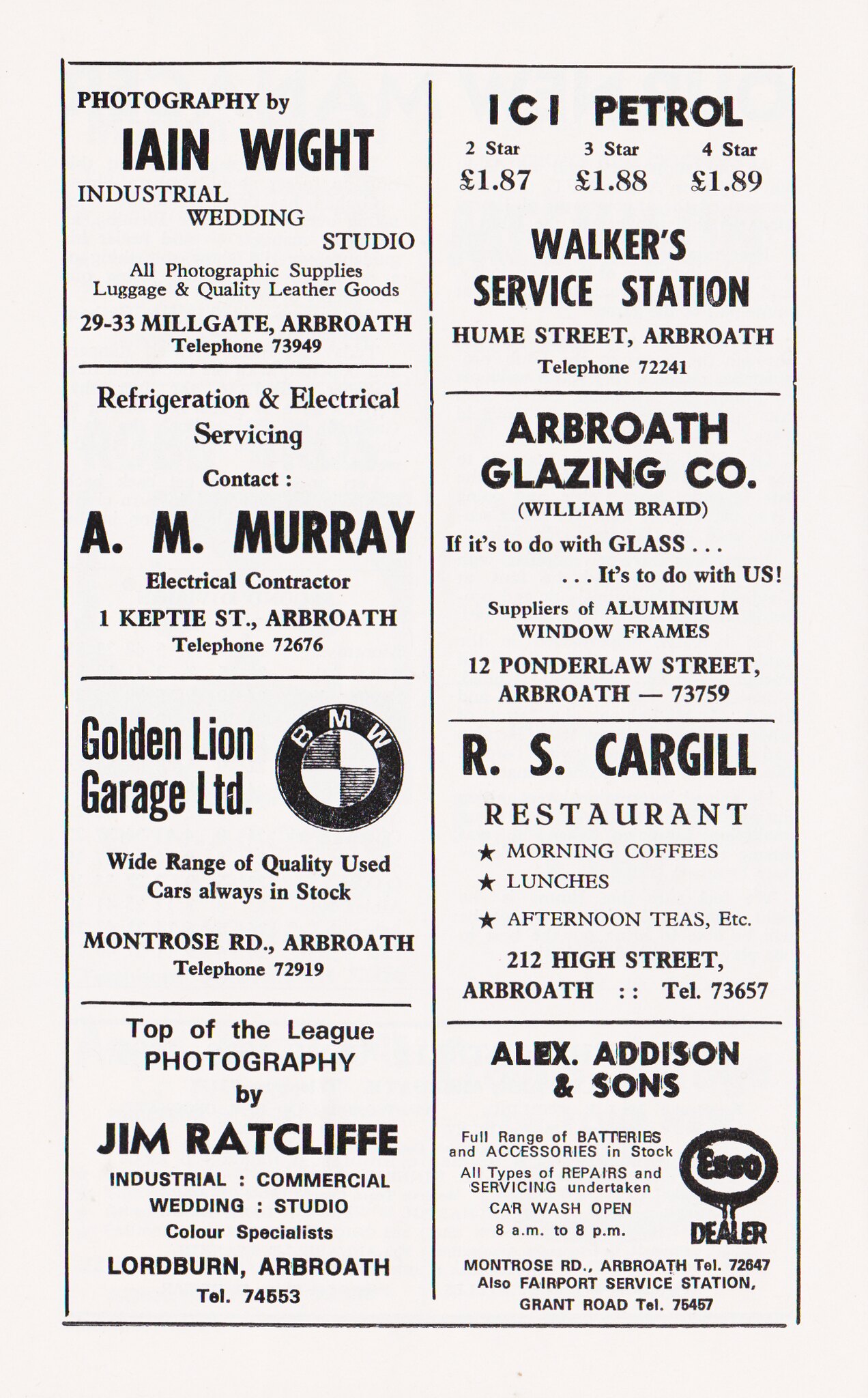This image depicts an advertisement section from a vintage publication, possibly from the 1960s or 1970s. The black and white page features eight advertisements arranged in two columns, each showcasing various local businesses. 

In the top left corner, there's a bold advertisement for "Photography by Ian Wright, Industrial Wedding Studio," located at 29-33 Middlegate, Arbroath, offering photographic supplies, luggage, and quality letter goods. Below it, another ad promotes "A.M. Murray" for refrigeration and electrical servicing.

Adjacent to these on the right, the topmost ad is for "ICI Petrol, Walker Service Station," followed by the "Arbroath Glazing Company." Further down on the left column, "Golden Lion Garage LTD" advertises next to the BMW symbol, and beneath it, "Top-of-the-League Photography by Jim Ratcliffe" offers additional photographic services.

In the adjacent right column, beneath the glazing company ad, is "R.S. Cargill Restaurant," inviting patrons for morning coffees, lunches, and afternoon teas. On the bottom right, "Alex Addison & Sons," an Esso dealer, completes the set of advertisements. The entire layout suggests this could be a sponsor page from a community event program, emphasizing its local business support.